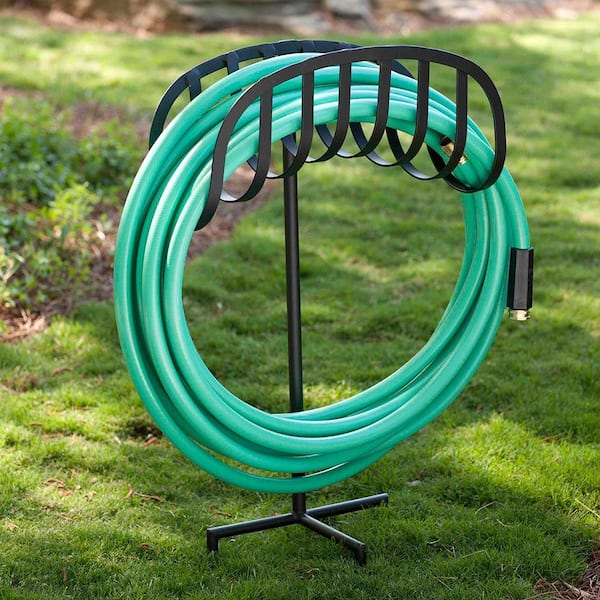The image portrays a well-maintained, vibrant green lawn, with some patches of brown showing through. On the left side of the lawn, there is a small garden area featuring green plants emerging from dark soil and some mulch, accompanied by bushes and rocks. Dominating the center foreground, a black metallic hose holder is securely anchored into the grass with three pronged legs. The stand supports a long vertical rod that curves into a top section designed with coils to hold a garden hose. Wrapped neatly in circular loops around the holder, the green garden hose features a black handle and a gold spout at its visible ends. The photograph, taken outdoors in broad daylight with ample natural light, is bright and clear, though the background becomes slightly blurry towards the middle and top portions of the image. The overall clarity of the hose and its holder is sharp, emphasizing the gardener's readiness for watering tasks.